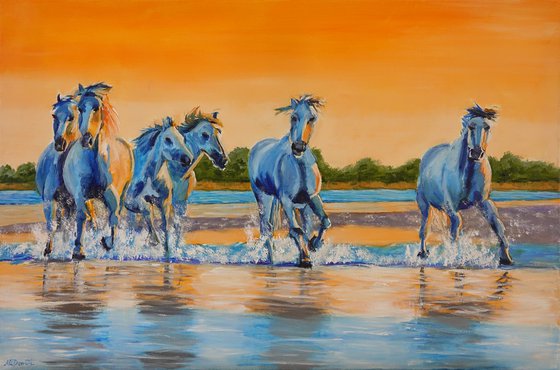A computer-generated art print depicts six wild, white horses running through shallow water under a vibrant, orange-gold sky. The sky's saturation decreases gradually towards the horizon, blending into a pale, whitish-yellow hue near a distant tree line. The water reflects the warm hues of the sunset, capturing the movement of the horses as they gallop, their manes flowing and knees bent. The scene is set with a backdrop of faint green trees or shrubs. Water splashes around their ankles, highlighting the playful and expressive nature of the horses enjoying a serene moment in a colorful and slightly abstract setting. No people or buildings interrupt the natural beauty of this unspoiled landscape.